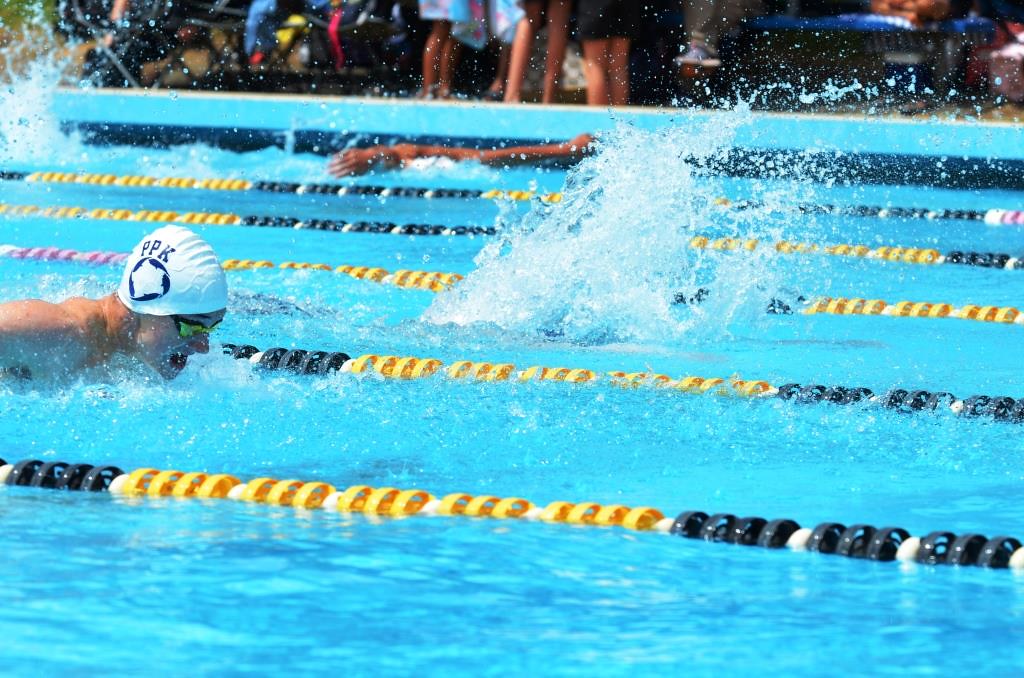This photograph captures a dynamic scene of a swimming race, prominently featuring a pool with floating lane dividers in white, navy blue, and bright yellow. The pool lanes are bustling with swimmers, distinguished by their white swim caps emblazoned with "PPK" in blue letters and a blue and white circle, and their water goggles. Splashing water is abundant, adding to the intensity of the race. In the upper left-hand corner of the image, one swimmer is particularly noticeable, their mouth open as they prepare to re-enter the water, with a tan arm visible mid-stroke. The background is filled with spectators, though only their legs are visible, hinting at the crowd's presence and their attentiveness to the race.